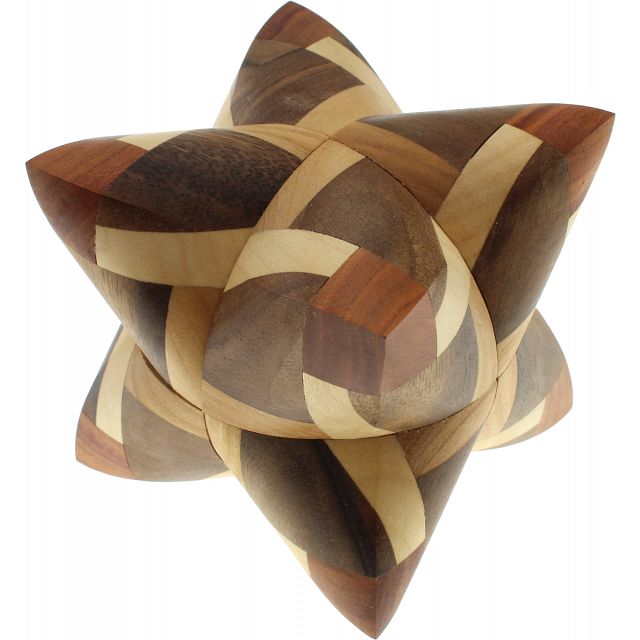This photograph displays a meticulously crafted, three-dimensional star shape set against a stark white background. The star is composed of seven pointed segments, resembling well-stuffed, triangular pillows. Each of these segments is formed from various types of wood, displaying a beautiful patchwork of light brown, medium brown, dark brown, cream, and golden hues. The wood's natural grain is clearly visible, enhancing the star's intricate design. The star is front-facing and sits prominently in the center of the image, showcasing its detailed construction and artistic flair. This piece, devoid of any text or signature, stands out as a striking artistic creation that blends together different textures and shades of wood into a cohesive, eye-catching decoration.